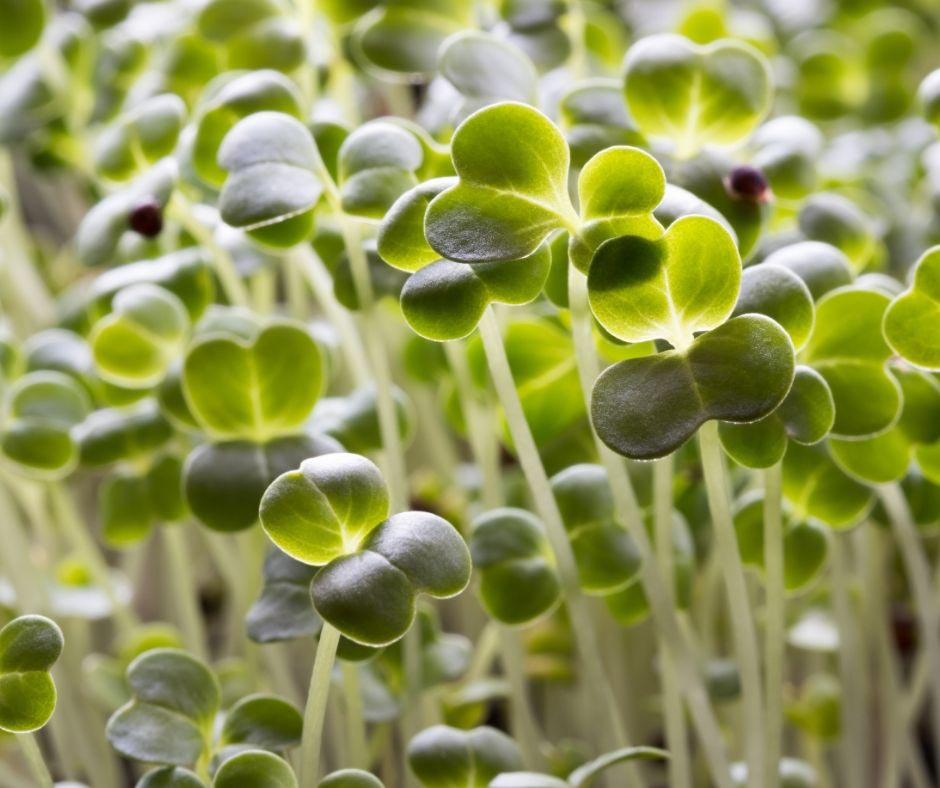This photograph captures a densely packed field of four-leaf clovers, each with subtle variations that hint at a possible variant of the typical clover. The image is a close-up, revealing hundreds of these green plants with their thin, translucent stems. The four green leaves of each clover reflect the sunlight differently, highlighting their veins and spines in some, while others appear as solid green without light penetration. The clover leaves at the bottom are notably darker than the lighter ones at the top, suggesting two distinct pairs. The background is entirely filled with clovers, leaving no ground visible and cutting off midway down the stems. A blurry, purple-colored bug can be seen clinging to one of the plants in the middle of the photograph, adding a touch of life to the serene scene.